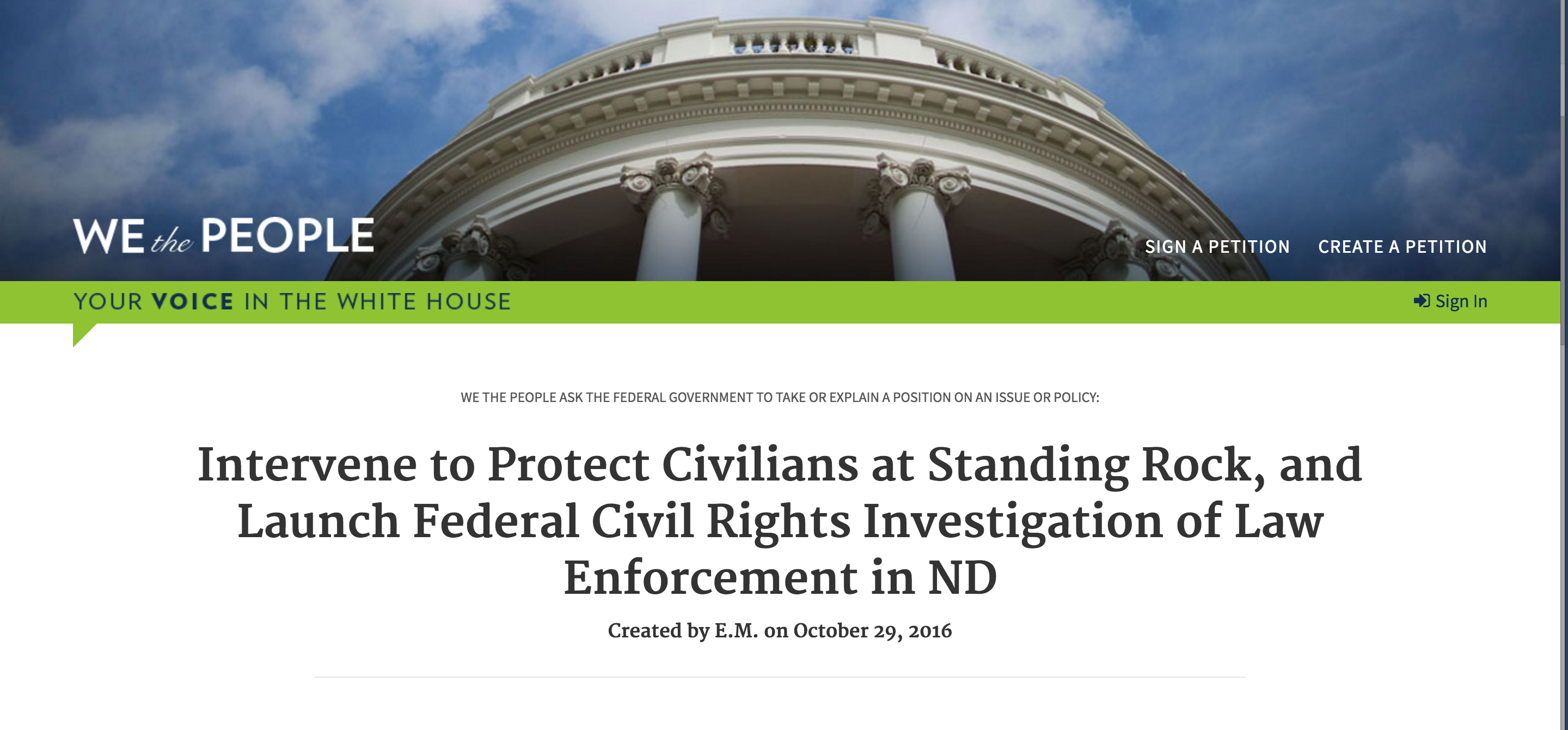The image depicts a webpage for a petition service with the White House featured prominently at the top, surrounded by blue, cloudy skies. Overlaying this image, positioned at the bottom, the phrase "We the People" is displayed on the right side, while on the left, prompts to "Sign a Petition" and "Create a Petition" are visible. Underneath this header, there is a green sign on the side that reads, "Your Voice in the White House."

Further down, text explains the purpose of the site: "We the People ask the federal government to take or explain a position on an issue or policy." Below this explanation, bold black letters announce a specific petition: "Intervene to protect civilians at Standing Rock and launch Federal Civil Rights Investigation of Law Enforcement in ND," attributed to a creator identified as E.M., dated October 29, 2016. This information is centrally located on the page, followed by a horizontal line close to the top of the image, with no further text below it.